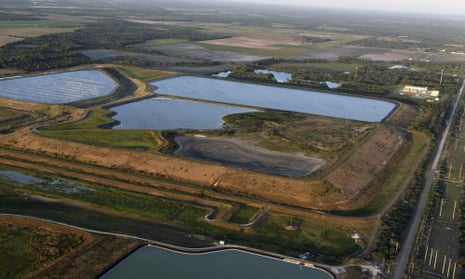This is an overhead aerial view of a rural countryside setting, likely taken professionally. Dominated by expanses of green fields and dotted with patches of brown and yellowish land, this area also features three distinct bodies of water. Centrally positioned and resembling small lakes or ponds, these water bodies include one with visible white lines whose purpose is unclear. An additional body of water can be seen at the bottom center of the image. A road traverses the scene from the bottom right, meandering towards the right side of the picture. The landscape is interspersed with fields, trees, and some small white structures that may be buildings, though they appear too small to identify clearly. The absence of visible vehicles and people, combined with the presence of a telephone pole, suggests a sparsely populated, non-residential area, perhaps farmland. The sky at the top edge of the picture is a dull grey, indicating daylight. The color palette of the image includes shades of green, blue, white, yellow, brown, gray, and a touch of orangish hues, reflecting the natural and somewhat industrial elements of this rural landscape. In the distance, mountains are faintly visible, adding to the scenic yet utilitarian character of the area.